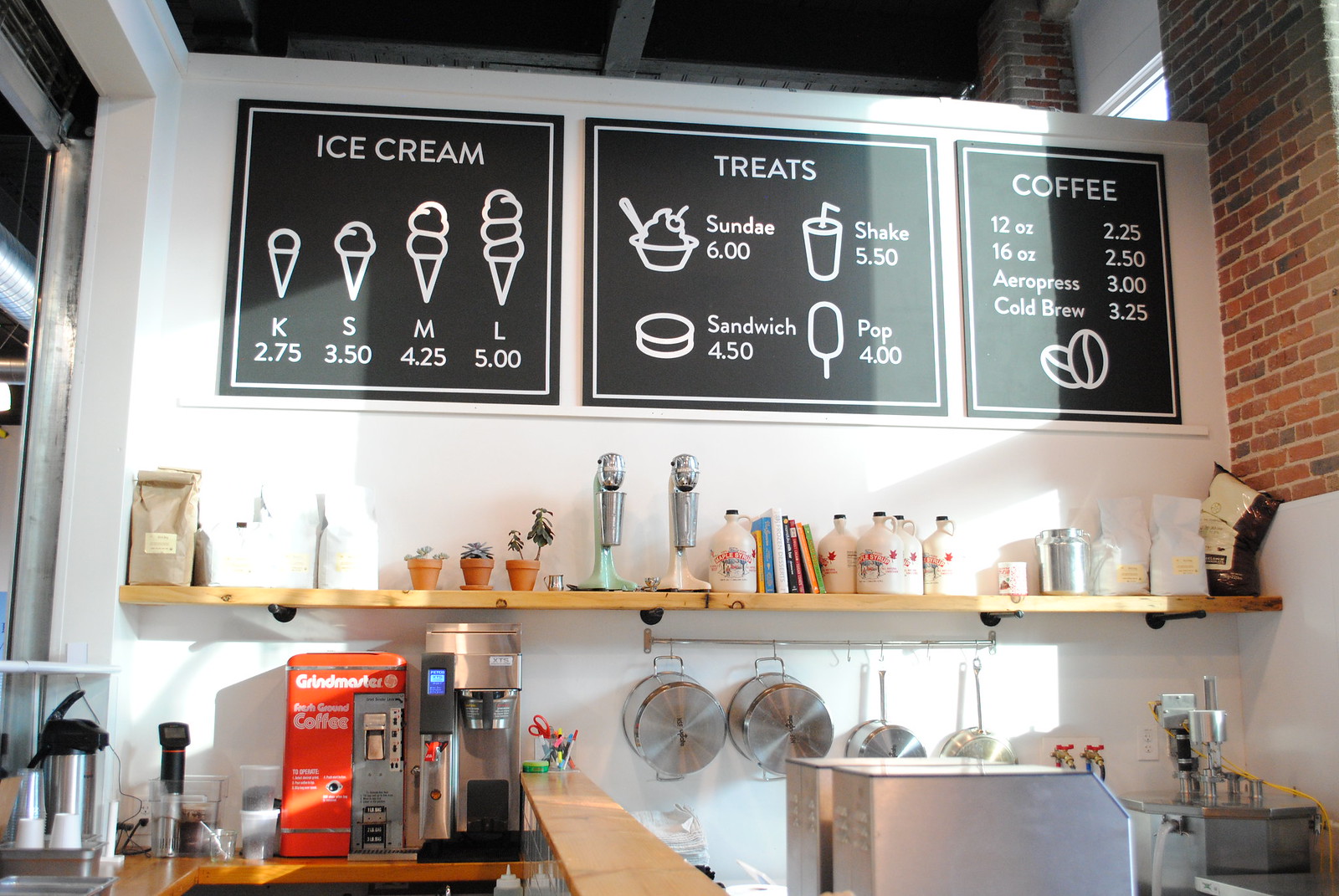The photograph, taken in full color during the day inside an ice cream shop that also sells coffee, showcases a detailed view of the back wall and menu. The back wall is white and adorned with three blackboards acting as the menu. The first menu on the left is labeled “Ice Cream” and lists four sizes with their prices: Kids $2.75, Small $3.50, Medium $4.25, and Large $5.00, each accompanied by pictures of ice cream cones. The middle menu, labeled “Treats,” offers a sundae for $6.00, a shake for $5.50, a sandwich for $4.50, and an ice cream pop for $4.00. The right menu, under “Coffee,” lists various coffee options: $12.00, $2.25, $16.00, $2.50, espresso $3.00, and cold brew $3.25. Below these boards, a wooden shelf holds two milkshake mixers, three potted plants in terracotta pots, multiple large jugs of maple syrup, and an assortment of kitchen utensils including paper bags, an orange coffee grinder, and a coffee maker. Light shines through a window on the upper right side of the red brick wall, illuminating the scene.